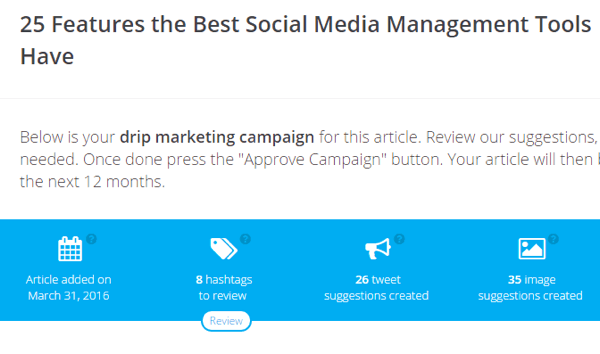The image features a white, horizontal rectangular banner with black text that reads "25 Features the Best Social Media Management Tools Have." Below this, there is a light gray, horizontal dividing line. 

Following the line, a bold, black font statement declares, "Below is your drip marketing campaign emphasis on this." It continues with details in a standard font, "For this article, review our suggestions needed. Once done, press the 'Approve Campaign' button. Your article will then [be live] in the next 12 months."

Beneath this section, a blue horizontal rectangle appears with white text. This section is filled with various icons and text including:
- A calendar icon with the text, "Article added on March 31st, 2016."
- Icons indicating arrows with the text, "8 hashtags to review" alongside an option to review.
- A megaphone icon with the text, "26 tweet suggestions created."
- A landscape photo icon noting, "35 image suggestions created."

Each text is accompanied by small circled question mark icons in a grayish color at the top right, which could provide additional information or tooltips when interacted with.